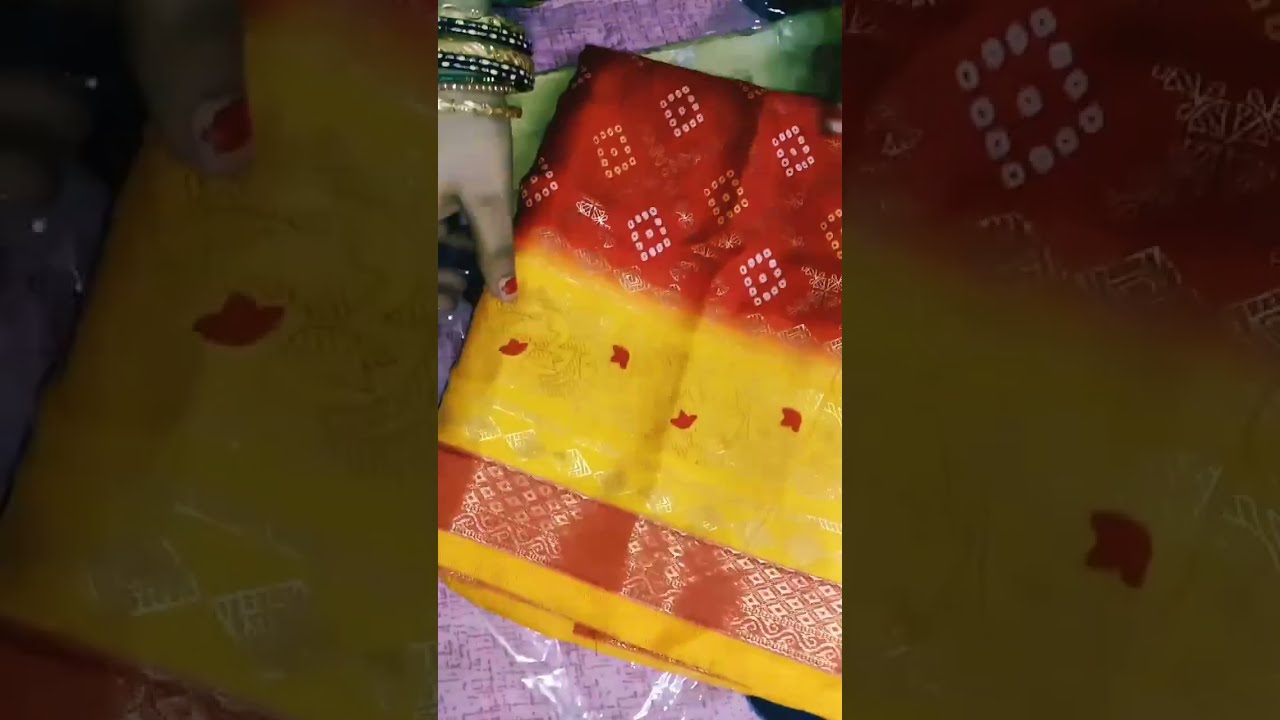This detailed image captures the right hand of a person with an Indian skin tone, adorned with numerous bracelets, primarily in gold and dark green, with a few featuring multicolored jewels, especially green ones with white dots. The person has chipped pink nail polish on their thumbnail, which is about 75% worn off. Positioned in the upper left-hand corner, the hand reaches down to grasp a folded piece of fabric with intricate patterns.

The fabric, potentially a silk scarf, is elaborately designed with sections of red, yellow, and a hint of purple, light green, and pink beneath it. The top red portion features diamond shapes formed by white symbols, including circles and squares, interspersed with floral designs. Below this, a bright yellow section displays red flying birds and silver embroidery, creating a vibrant contrast. Further down, a thin lighter red stripe is adorned with silver diamond patterns and squiggly lines. At the very base of the fabric, there is a decorative pink trim with shiny pink diamonds. The overall composition suggests a display piece, possibly in a department store setting, emphasizing the rich and colorful textile artistry.